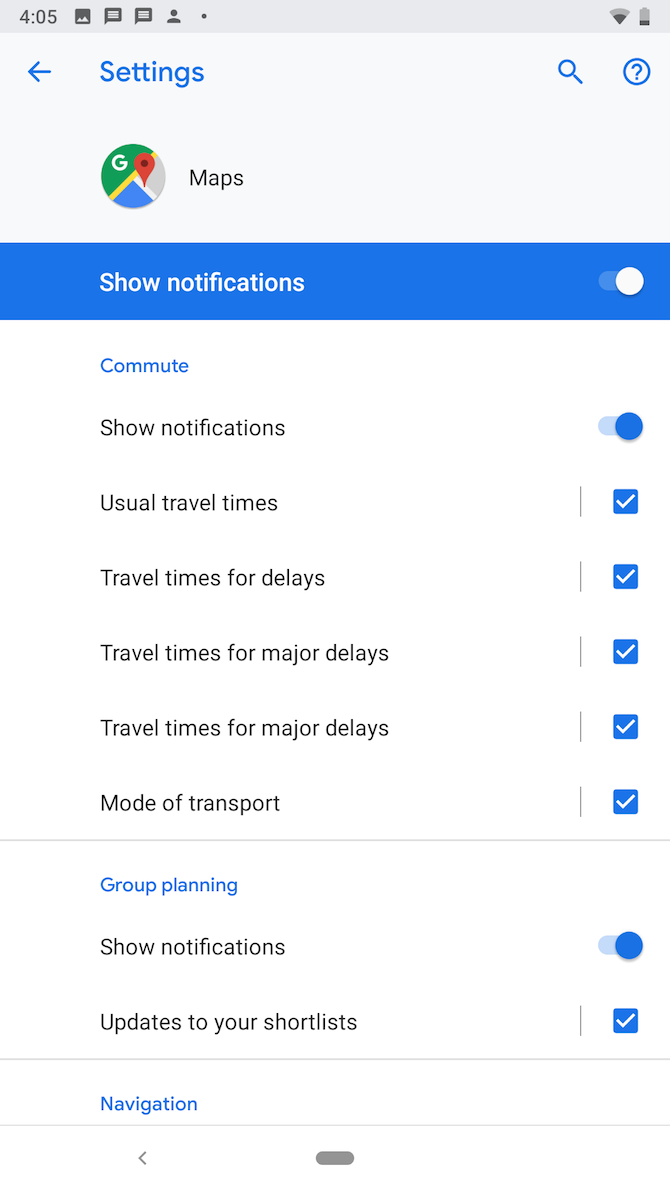In the image, the top left corner displays the time as 4:05. Adjacent to this, icons for various functions are visible including a speaker for volume control, a left arrow, the word "Settings," a small magnifying glass for searching, and a question mark inside a circle. Right next to these icons is the option for Google Maps.

Beneath these options, there is a section labeled "Show Notifications," with a toggle switch positioned to the right, indicating that notifications are enabled. Below this, the text “Commute” appears in blue. Under the "Commute" category, multiple options are listed with their corresponding settings:

- "Show Notifications" is enabled with a blue toggle switch to the right.
- "Usual Travel Times" has a checkmark inside a blue square.
- "Travel Times for Delays" is checked.
- "Travel Times for Major Delays" is checked twice, each with a blue checkmark.
- "Mode of Transport" is checked.

Further down, the section labeled "Group Planning" in blue text appears. Under this category, there is a "Show Notifications" option with the toggle switch shifted to the right, represented by a blue circle. The "Updates to Your Shortlists" option is checked, indicated by a blue box with a checkmark.

Finally, the bottom of the image contains the word "Navigation."